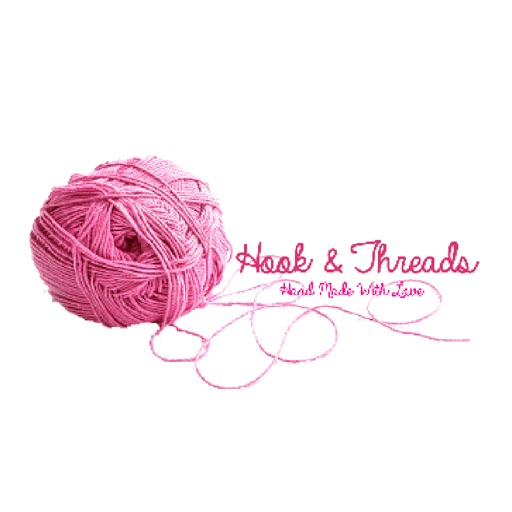This horizontal image, set against a pure white background, features a prominently positioned ball of bright pink yarn. The yarn ball appears slightly unraveled, with loose threads curling out and sprawling around the image, particularly beneath the text on the right. The yarn, possibly woven from wool or similar fibers, is wrapped in various directions, with a hole in the center suggesting it was wound around a post or knitting needle. Accompanying the yarn is pink cursive text that reads "Hook & Threads" in a bold, elegant script. Below this, in a smaller cursive font, is the phrase "Handmade with Love". The overall image has a slightly grainy, blocky quality, with particularly rough edges around the free strand of yarn.